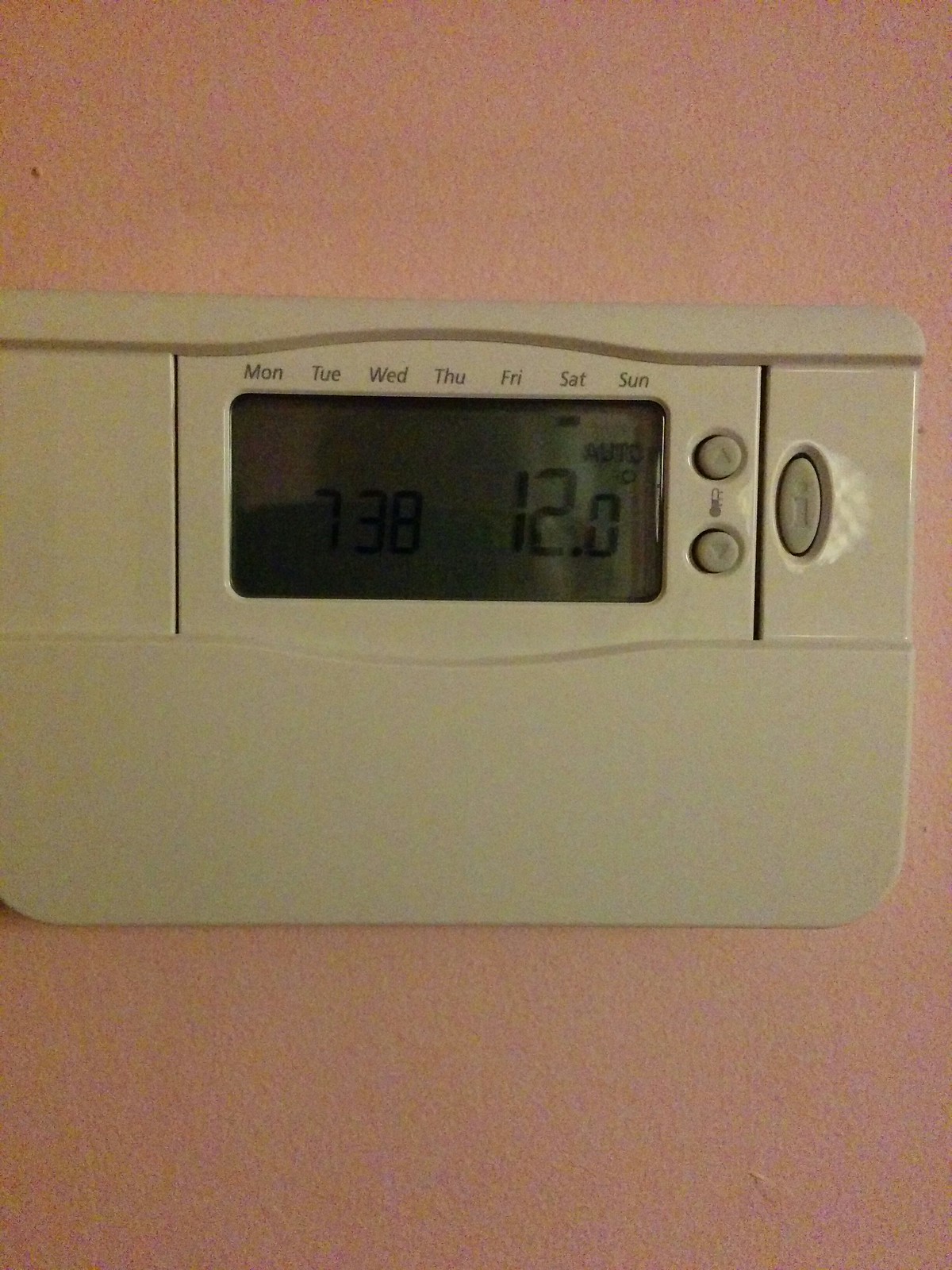A digital photograph, taken inside a house, features primarily a white digital thermostat mounted on an off-white, slightly textured wall. The wall spans the entire width of the image, from left to right. The off-white wall, with its subtle raised bumps, provides a neutral backdrop to the prominently displayed thermostat.

The thermostat itself is an almost square-shaped, rounded-rectangle device. Its intricate design includes a top edge with a thin line that dips towards the center, rises, and then levels off as it extends to the right. Centrally located, a vertical slit adds to its detailed architecture, paralleled by another slit on the right edge.

Dominating the top section of the thermostat is an old-style LCD screen. In gray print, the abbreviations for the days of the week (MON, TUE, WED, THU, FRI, SAT, SUN) are clearly visible. The screen is split with the left side displaying "7:38" and the right side showing "12.0°C" with a small, raised degree symbol, indicating the temperature in Celsius. Above the temperature readout, the word "AUTO" is displayed prominently in capital letters.

Adjacent to the LCD screen are two small gray buttons: an up arrow on the top button and a down arrow on the bottom button, used to adjust settings. Below these buttons is an old analog display gauge, which further emphasizes the thermostat’s hybrid design of digital and analog features. A horizontal line separates these elements from an oval, vertically oriented button marked with a lowercase "i" embedded in a small indent.

This meticulously designed thermostat harmonizes form and function, standing out against the textured wall backdrop to offer precise control over the household temperature.